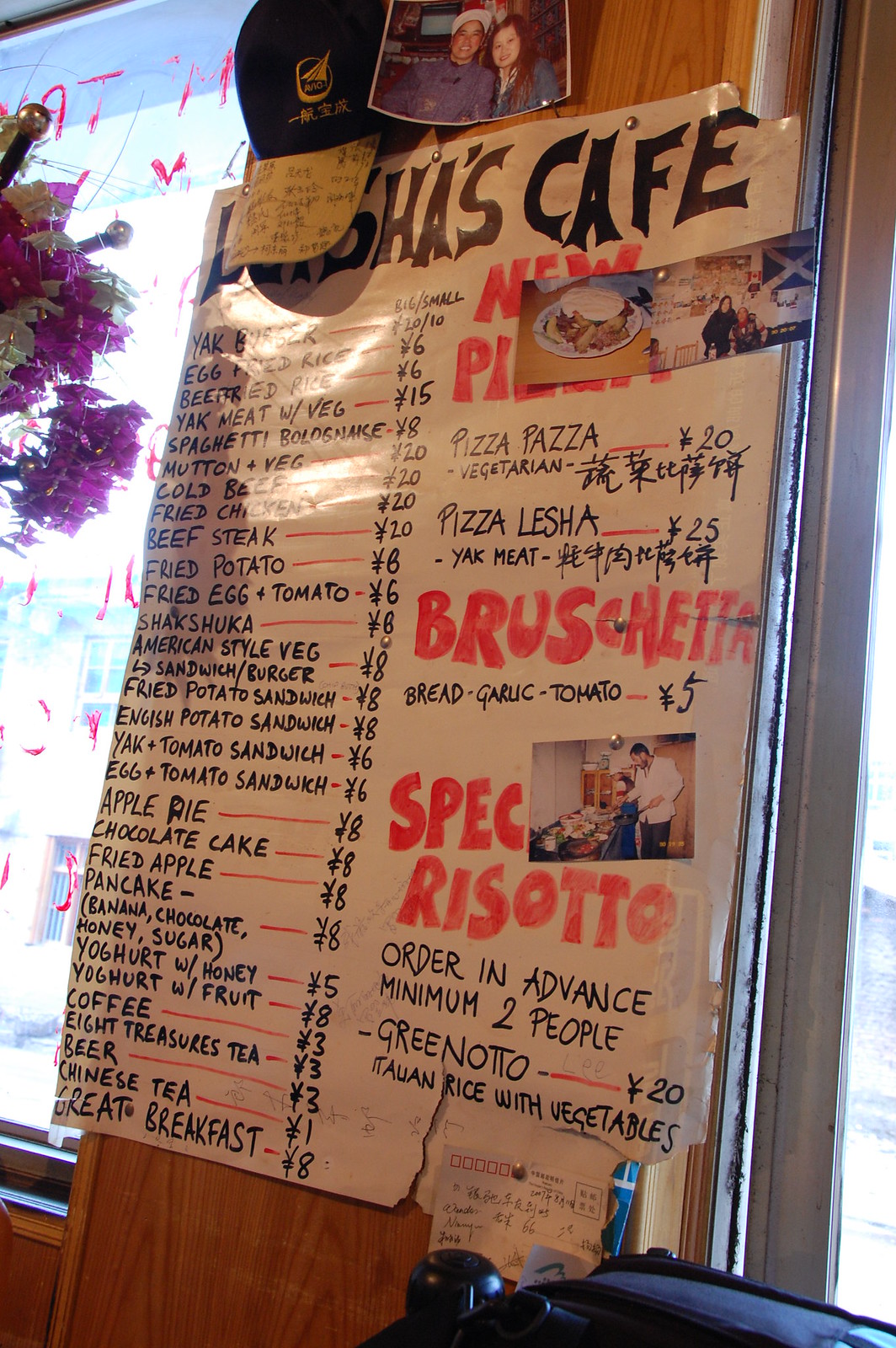The image is a portrait-format photograph taken by either a phone or a camera, depicting a menu pinned to a wooden wall between two windows. The menu is slightly tilted, extending from the upper right corner to the lower left corner. At the very top of the menu, there's a picture of a man wearing a Santa hat and a woman standing next to him. To the left of this picture, a black ball cap with a cream brim is signed on the brim, obscuring part of the cafe's name, though the word 'Cafe' is clearly readable.

The menu itself is white and laminated. It's divided into two halves: the left half lists various food items in a long column with red lines connecting the items to their respective prices. These items include yak burger, egg fried rice, beef fried rice, yak meat with vegetables, spaghetti bolognese, mutton with vegetables, cold beef, fried chicken, beefsteak, fried potato, fried egg and tomato, shakshuka, and several types of sandwiches, pies, cakes, and pancakes, along with drinks like coffee, tea, and beer.

The right half of the menu features items in larger print, with some listed in bold red and black text, such as bruschetta, special risotto (available by advance order for a minimum of two people), pizza, pasta, and vegetarian dishes. There are also pictures of food items and patrons pinned alongside the menu.

To the left of the menu, a window with red writing and purple flowers is visible, and sunlight streams through the windows on either side. The overall arrangement creates a cozy and inviting atmosphere, highlighting a diverse menu that hints at a blend of international and local cuisine.